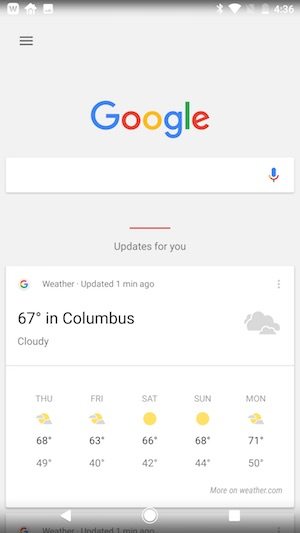This screenshot appears to be from an Android phone. The top of the screen features a subtle gradient transitioning from black to a light gray, the primary color of the screen. At the very top are several status icons: a "W" in a white box, a home icon, an image icon, a Bluetooth icon, a Wi-Fi symbol, a battery icon, and the time displayed as 4:36.

Below the status bar, on the left side, there is a hamburger menu icon (three horizontal gray lines). Centered at the top third of the screen is the Google logo, below which lies a white search box with a microphone icon inside, indicating a voice search option.

Underneath the search box, a small red line and the text "Updates for you" in gray are displayed. The screen then shows a white box containing weather information. The box includes a Google logo, the word "Weather" in gray, "Updated 1 minute ago," and an icon of three vertical dots indicating additional options. The current temperature is shown as "67°F in Columbus" with a "Cloudy" description in gray text.

To the right of the current temperature, cloud icons give a visual representation of the weather. A light gray line divides this section, followed by a forecast for upcoming days:

- **Thursday**: A sun icon with clouds, 68°F high, 49°F low
- **Friday**: Same sun and clouds icon, 63°F high, 40°F low
- **Saturday**: Sun icon, 66°F high, 42°F low
- **Sunday**: Sun icon, 68°F high, 44°F low
- **Monday**: Sun icon with clouds, 71°F high, 50°F low

At the bottom of the weather box, the text "More on weather.com" appears in gray. At the very bottom of the screen are three navigation icons: a back arrow, a circle (home button), and a square, all in white.